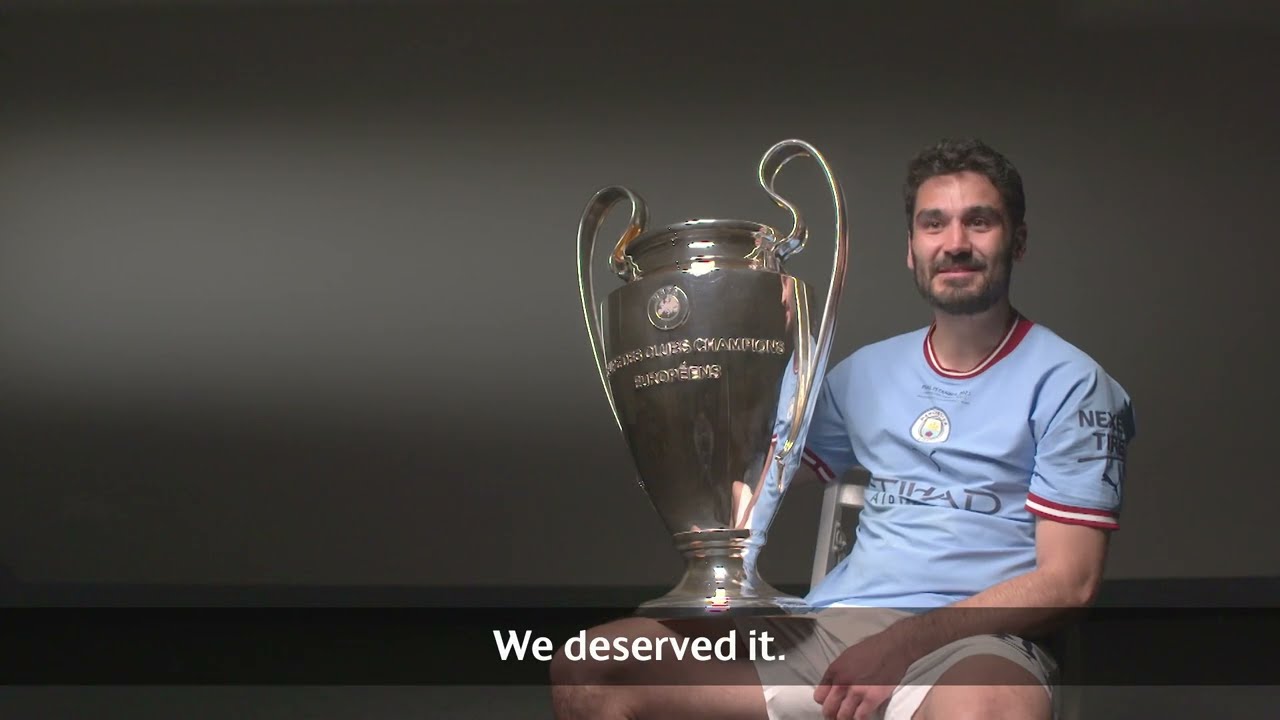In the image, a light-skinned man with short, dark brown hair sits in a silver metal chair against a dark, shadowy backdrop. The background, featuring an off-white wall, is dimly lit with a light reflection visible on the left side. The central focus of the image is a large, shiny gold trophy, shaped like a chalice with two ornate handles curving upward and then back down to the bowl. The trophy is positioned prominently on the man’s right leg, supported by his right hand.

The man is wearing a light blue sports jersey adorned with white bands and red stripes along the neckline and arm cuffs. He pairs this with white shorts, giving the impression of a sports uniform which suggests sponsorship branding. He has a thin mustache and beard stubble, and his expression shows a mix of happiness and pride with a subtle smile.

The man’s left arm and hand drape casually over his left leg, adding to his relaxed demeanor. At the bottom of the image, there is a darker gray bar with white text that reads, "We deserved it." The image captures a triumphant and celebratory moment, centered on the man's achievement symbolized by the impressive trophy.